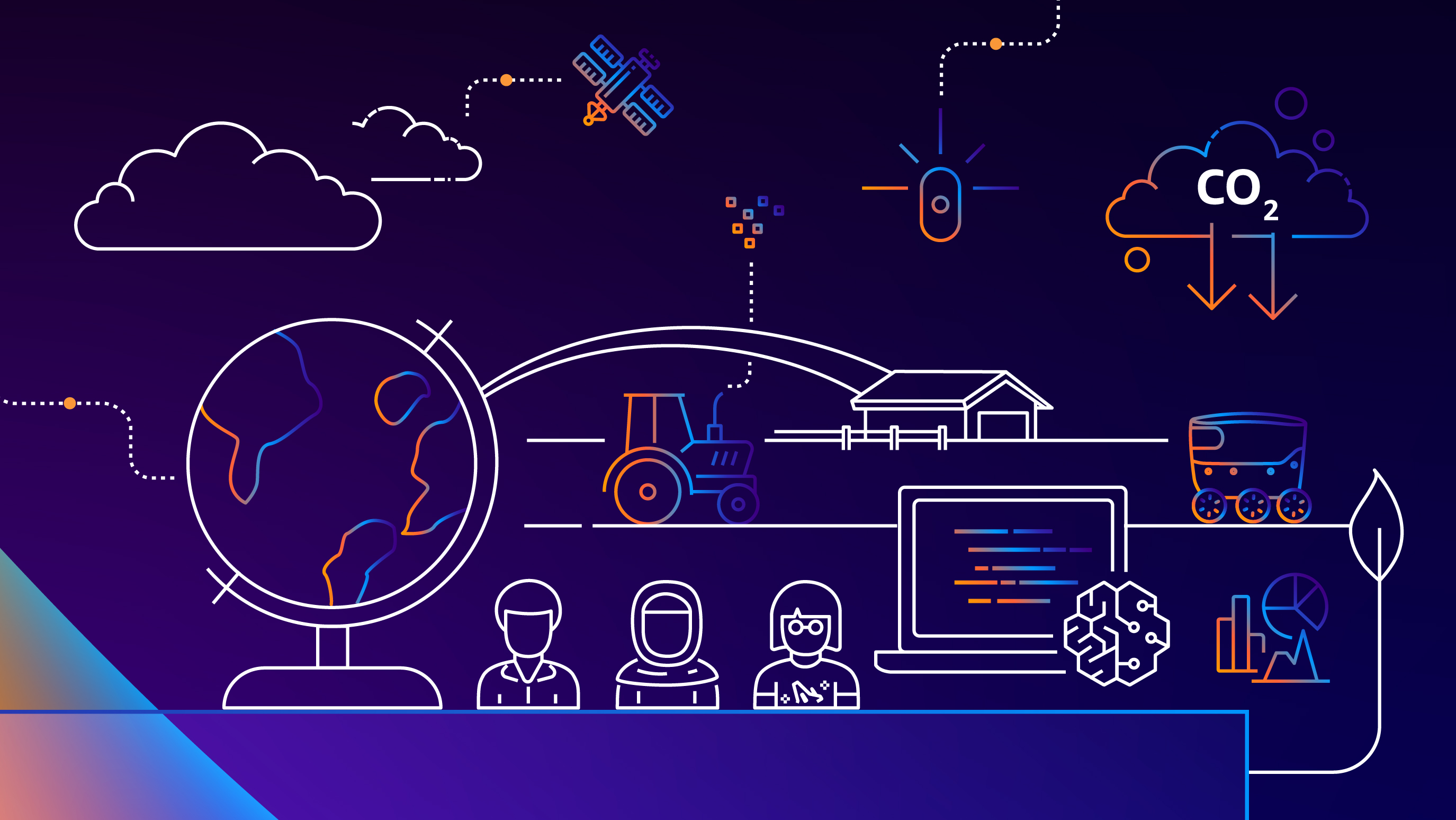This cartoon infographic features a long rectangular box with a dark to light purple gradient from top to bottom. In the lower left-hand corner, there's a triangle with a gradient from light blue to light pink. The infographic includes several elements: 

- White clouds, some containing dots leading to a purple, blue, and yellow satellite.
- Another cloud labeled "CO2" with arrows pointing down.
- A globe on the lower left connected to a farm scene, featuring a tractor emitting smoke.
- An old biplane flying among clouds and an oval representing the sun with sunbeams extending outward.
- A small trolley car depicted near the CO2 cloud.
- A computer displaying a brain with various graphics nearby.

Three figures, outlined mostly in white and shaded in purple, blue, and orange, sit at a table in the bottom section of the infographic.

This visual blend uses a colorful gradient and detailed illustrations to convey complex concepts, possibly related to environmental impact or technological progression. The collage vividly combines elements from space, nature, and technology, creating a layered and engaging visual narrative.